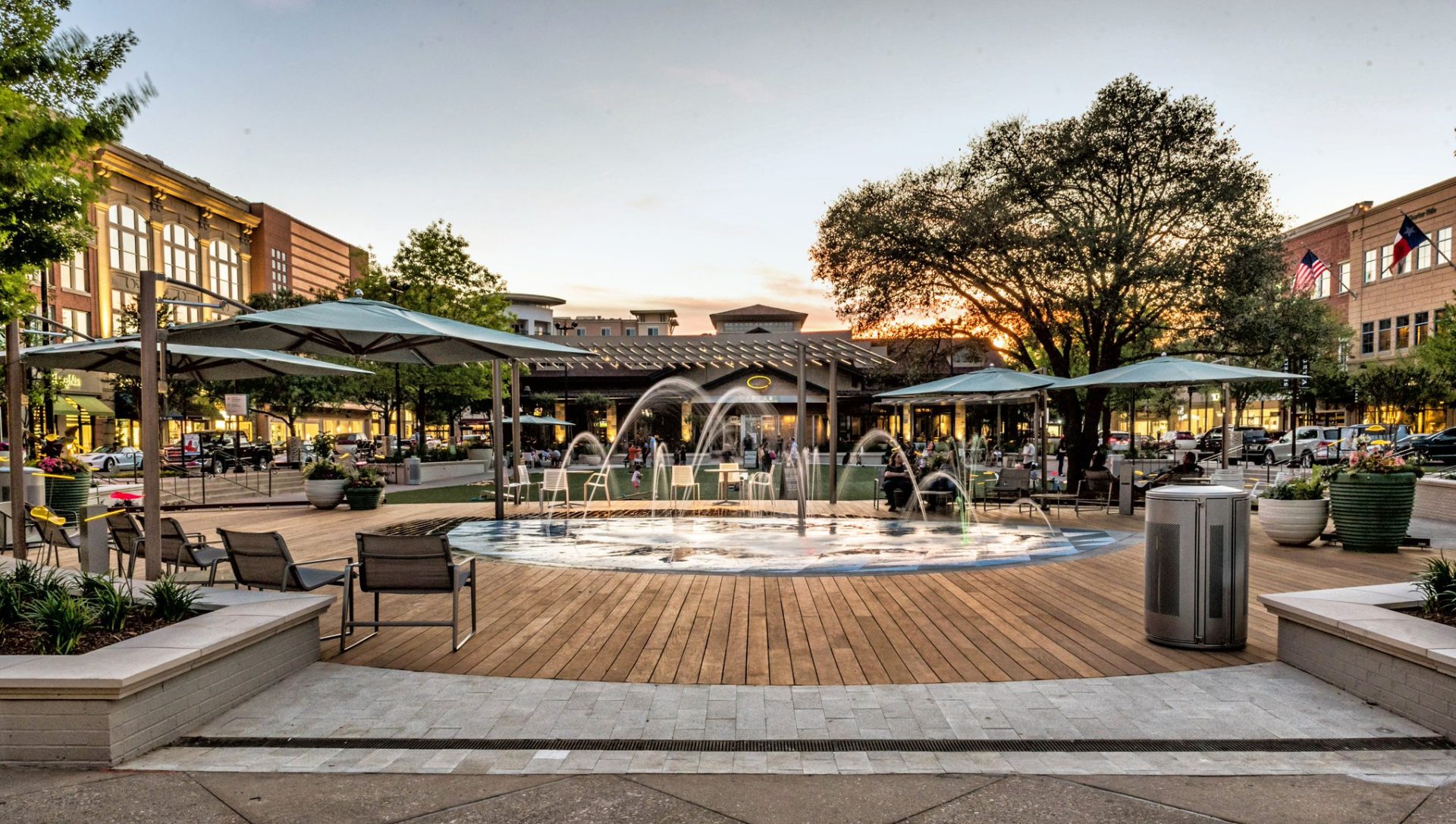This photograph depicts a charming small city park located in the middle of a bustling town, featuring a diverse blend of historical and modern elements. The foreground showcases a gray brick stone walkway leading to a circular wooden deck of a lighter brown hue, arranged with numerous outdoor chairs. Dominating the center of this deck is a striking fountain, with seven arcs of water gracefully shooting upwards. On the periphery, four dark blue-topped canopies house wicker benches, some of which are occupied by a few people toward the back right. The background is framed by lush greenery, including a tall, leafy tree to the right, while to the left and right, various buildings stand, including renovated older shops and newer glass-front stores. An American flag and a Texas flag adorn the right side, adding a patriotic touch. Above, the sky glows with the warm hues of a setting sun, casting a golden light across the serene and inviting scene.